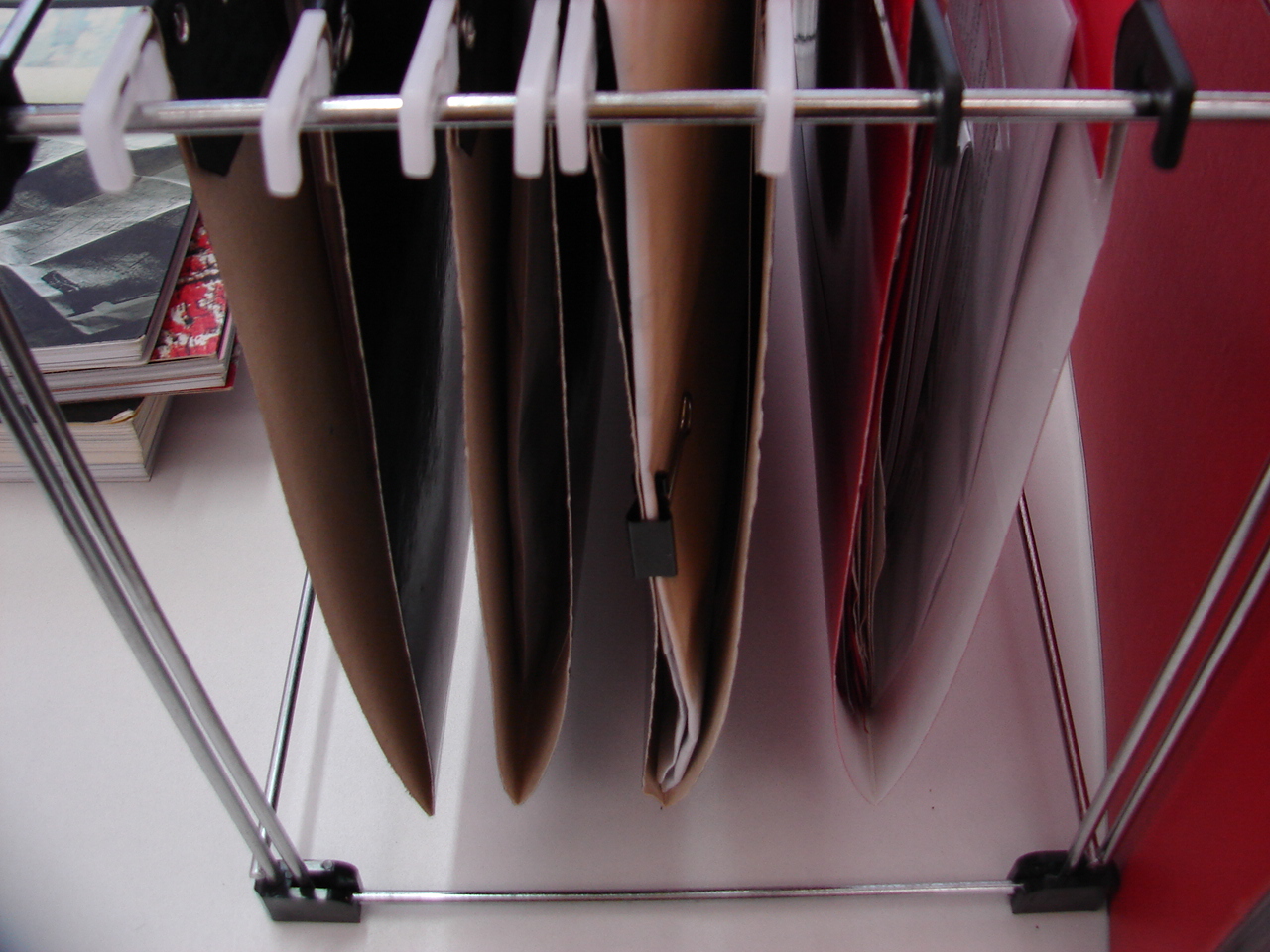The image depicts a close-up view of a desk organized with a folder holder. The holder consists of four metal poles serving as a frame, with white plastic hooks suspending the folders neatly as if in a binder. There are four folders attached: two on the right filled with papers, and two on the left remaining empty. The structure's base is framed with black connectors holding the silver wires together, while the top features a single wire from which the folders hang. The desk itself is white, and in the background, the right side reveals a hint of a red wall. To the left side, there are three books or notebooks stacked, though their exact nature isn't clear due to the focus on the folders. Notably, while most hooks are white, the last two are black, adding a unique visual detail to the setup.